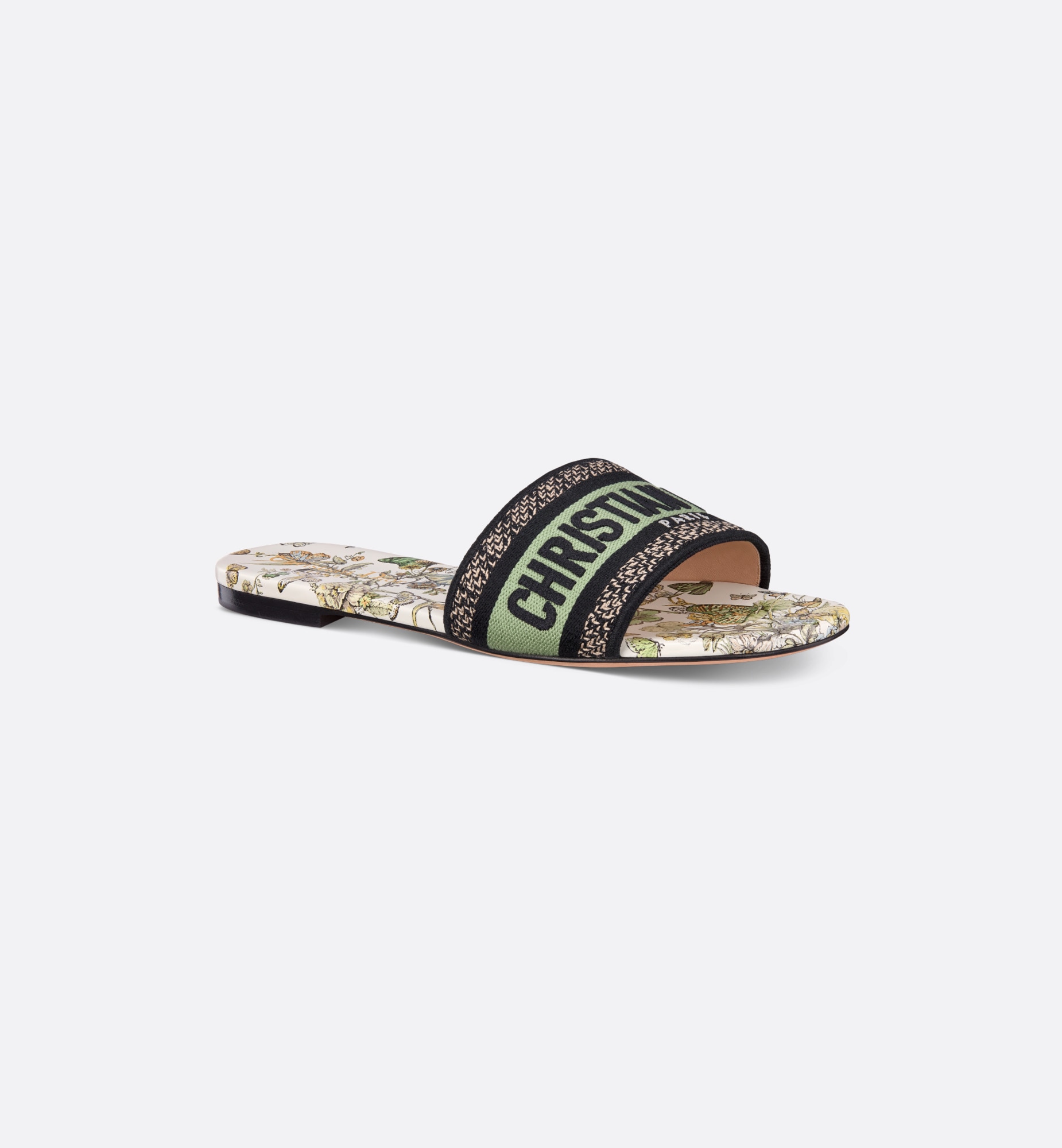This detailed color photograph features a single Christian Dior sandal set against a light grayish background. The sandal showcases a distinct low black heel, approximately a centimeter or a quarter inch in height. The footbed of the sandal is ivory or cream-colored, adorned with a green leaf floral print. The sandal has an open-toed, slip-on design characterized by a wide band that secures over the top of the foot. This band is bordered with black edges that feature a subtle white brocade pattern. Centrally, the band includes a light green strip of fabric, embroidered with the name "Christian" in brown or black text. The overall design is simple yet classically elegant, making it a stylish summer item that appears to be in pristine, unused condition.